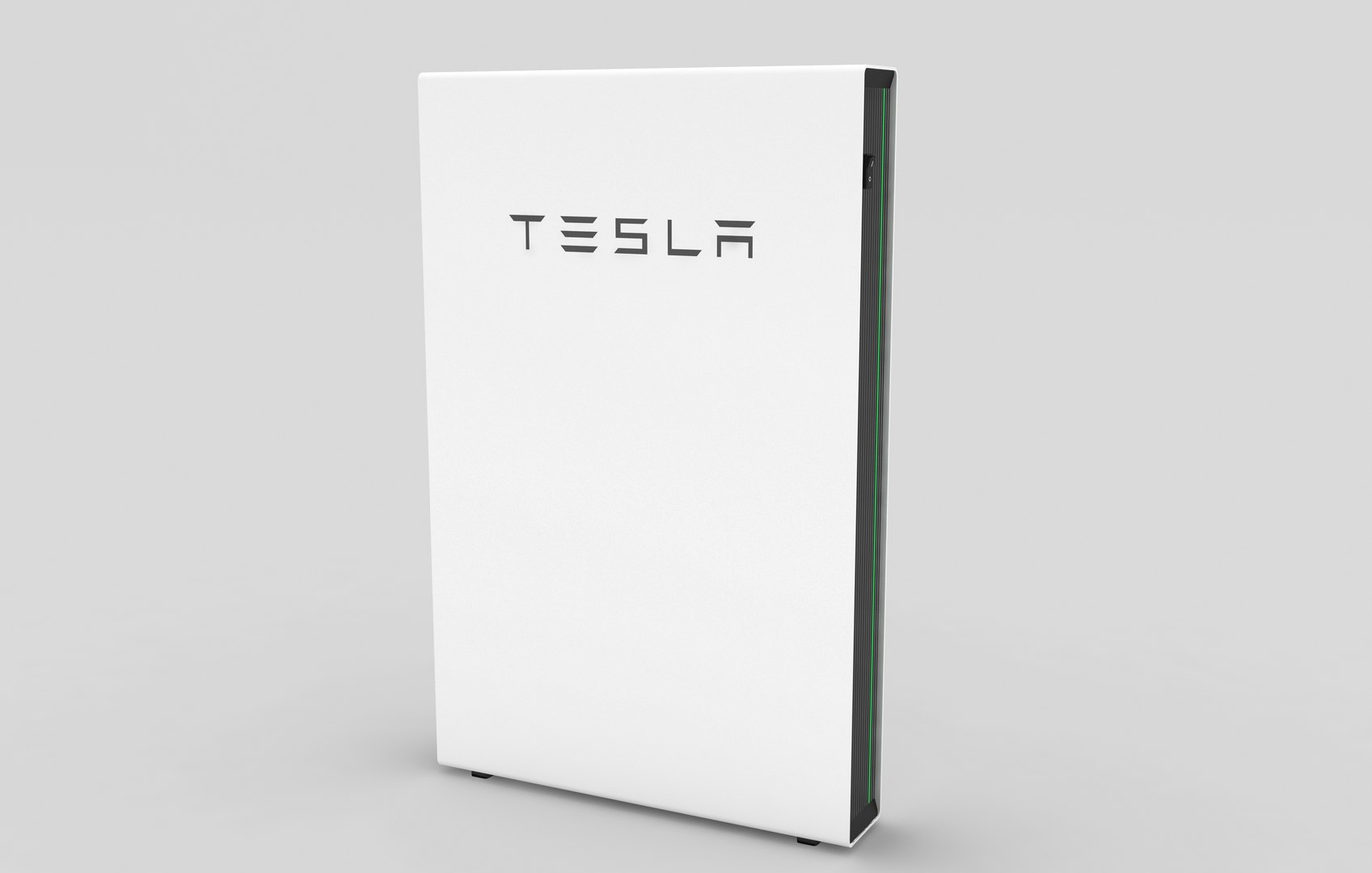The image depicts a sleek, white device that closely resembles the form factor of modern gaming consoles such as the PlayStation 4 or Xbox, standing upright. Featured prominently near the top, just off-center, is the Tesla logo in bold black lettering. The background is a neutral gray, which accentuates the device's clean lines and minimalistic design.

The device stands on two small, black feet located at its base, which provide support and elevate it slightly from the surface. On the right side, there appears to be an on/off switch, adding a functional element to its otherwise streamlined appearance. Subtle shadows to the left and right hint at its physical presence against the otherwise unembellished background.

Though the exact purpose of this device is not clear from the image, its aesthetic speaks to a modern, high-tech design ethos consistent with Tesla's brand.